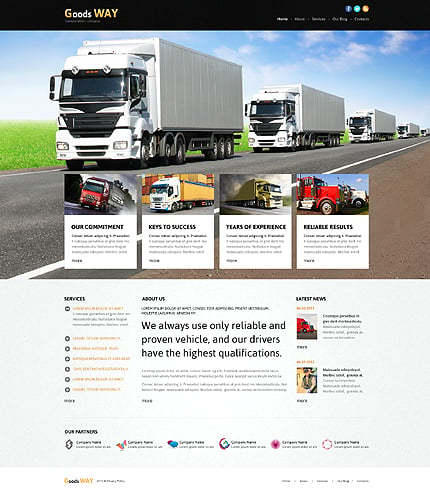This image depicts a screenshot from a company’s website, specifically for "Goods Way." In the upper left corner, against a black banner, the company name is displayed with the letter "G" in "Goods" being yellow and the rest of the text in white, while the word "Way" is entirely in yellow. In the far right upper corner, there is a blurry icon for Facebook with illegible text beneath it.

The central portion of the image features a color photograph showing a road with four semi-trucks, all white, driving towards the viewer in the same direction. This scene takes place beside a grassy field under a daytime sky that is blue with white clouds.

Directly beneath the main photo, there are four rectangular boxes, each containing an image of a different truck. From left to right, these boxes are labeled: "Our Commitment," "Keys to Success," "Years of Experience," and "Reliable Results.” The lower section of the image transitions into an area with a white background.